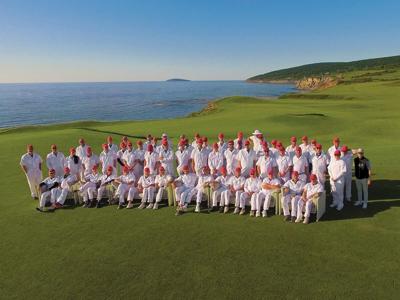In a low-resolution photograph taken from a slight elevation, a group of approximately 50 young men is gathered on a well-maintained grassy field, likely a golf course, positioned near a coastal cliffside with the ocean in the background. The men, organized in three rows—two standing and one seated in chairs—are uniformly dressed in red caps, white jerseys, and white pants. On the far right stands a man in a dark vest, tan pants, and a white hat, possibly a coach or manager. The backdrop features green rolling hills descending to the cliffs and a clear, blue sky devoid of clouds.